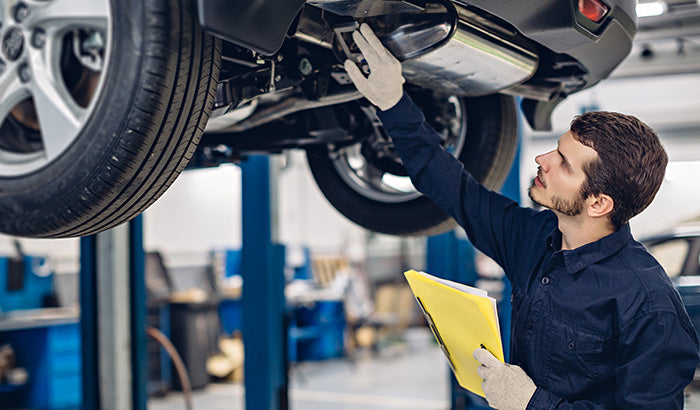In this horizontal color photograph, a mechanic is inspecting a car suspended on a lift within a blurred auto shop environment. The mechanic, positioned on the right side of the image, is a white male in his mid-twenties with brown hair, wearing a blue collared mechanic suit and white gloves. His right arm is stretched upwards, touching and examining the underside of the car, which showcases its two front wheels and extends from the upper left-hand corner to the right side of the image. In his left hand, partially down by his chest, he holds a yellow binder filled with papers. The background is a well-lit mechanic shop featuring indistinguishable, blurred elements including a blue car, metal poles, and various equipment against a white wall. The overall scene captures a focused moment of the mechanic diligently working on the vehicle.